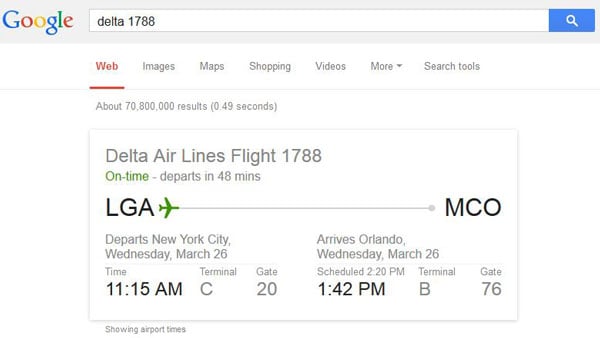**Detailed Caption for the Image:**

The screenshot displays the Google search results for "Delta 1788." The familiar Google logo, with its traditional color scheme of blue, red, yellow, green, and red letters, is prominently featured in the banner at the top. Below the logo is the search bar containing the query "Delta 1788." Various search options are listed beneath the search bar, including web, images, maps, shopping, videos, more, and search tools.

The search results indicate there are approximately 70,800,000 results found in just 0.49 seconds. A highlighted gray box provides pertinent flight details: Delta Airlines Flight 1788 is scheduled to depart on time in 48 minutes. The flight originates from LaGuardia Airport (LGA) in New York City and is destined for Orlando International Airport (MCO).

The specific flight timing and details are as follows:
- Departure from Terminal C, Gate 20 at LaGuardia (LGA) on Wednesday, March 26th at 11:15 AM.
- Arrival at Terminal B, Gate 76 at Orlando (MCO) on the same day, March 26th, at 1:42 PM.

Both departure and arrival times are noted in Eastern Time Zone. This detailed information indicates the flight duration and the logistics of the journey from New York City to Orlando.